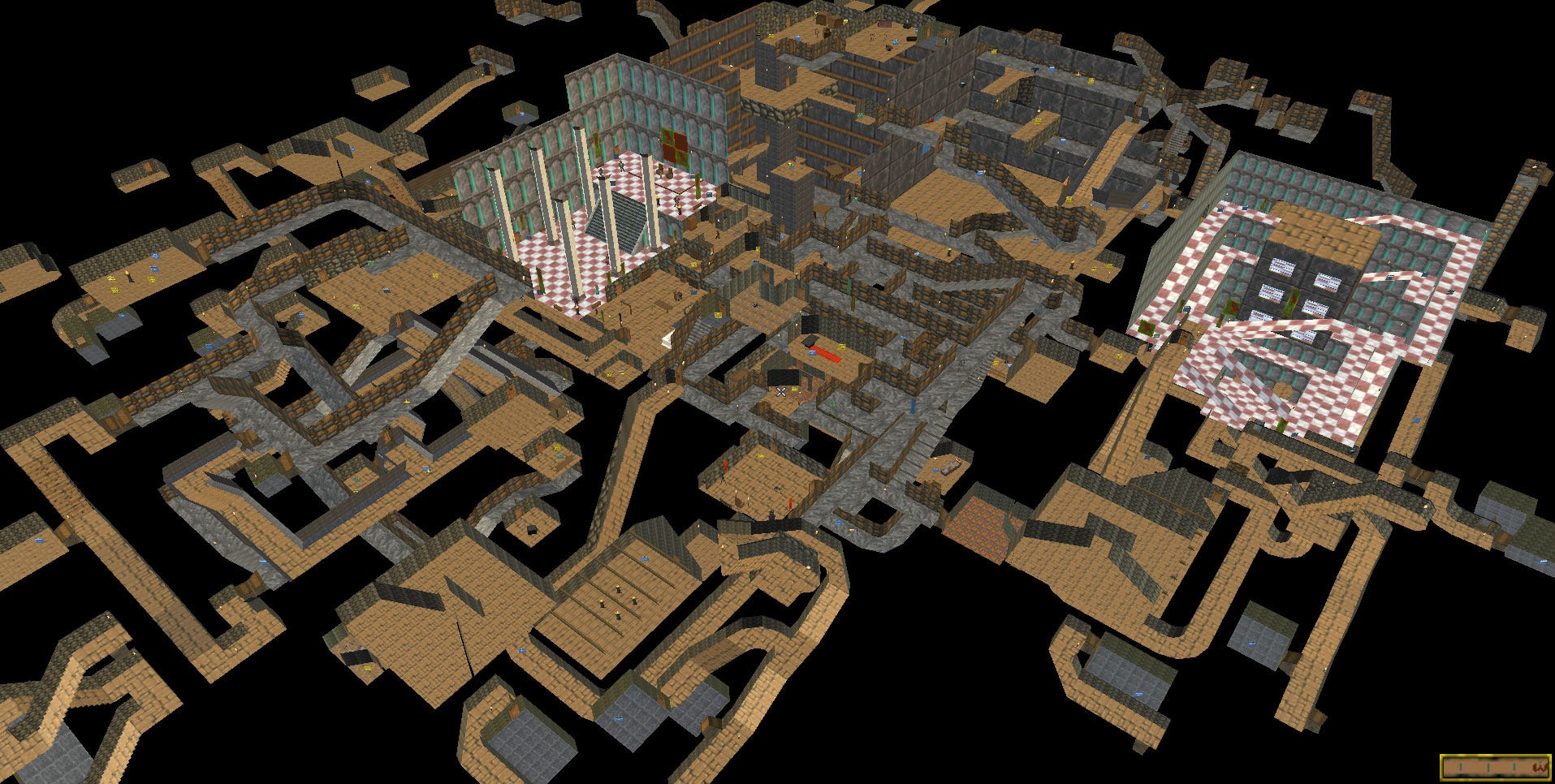The image appears to be a detailed computer-generated graphic, reminiscent of a video game design. The setting is outdoors with a predominantly black background, and it depicts the layout of what seems to be a town or a series of buildings. The structures are primarily composed of brown elements, giving them a blocky appearance similar to Minecraft or Lego formations. Notably, in the bottom right corner, there's a distinctive building topped with a red-and-white checkered pattern, which also appears on a wall and roof of a similar brown building in the middle of the image. Silver pillars and some green features are visible in the background, along with ramps leading to smaller buildings. The layout spans diagonally from the bottom left to the top right of the image. Scattered throughout are small figures, represented as black cylinders with white dots, and some red cylinders. Despite the detailed design, there is no readable text within the image.